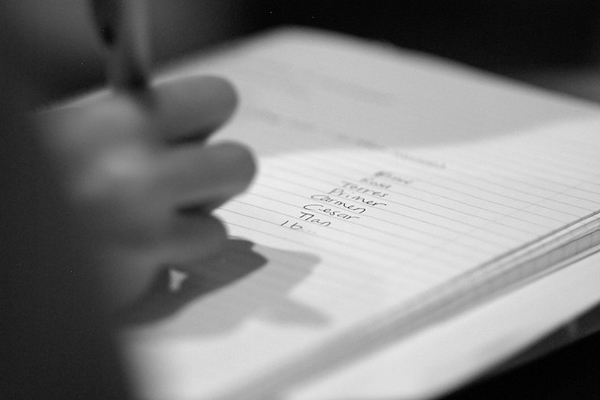A black and white close-up photograph captures a young person's right hand, slightly out of focus, clasping a pen or pencil as they write on a lined notebook page. The paper, which appears to be part of a ruled, possibly spiral-bound notebook, features a list of names, including "Primer," "Carmen," "Cesar," and "Tian" or "Nan," followed by "1B." The background of the image is dark and blurred, bringing subtle emphasis to the notebook's lines and the partially legible writing on the paper. The overall image has a blurry, unfocused quality, especially around the borders, drawing attention to the central activity of writing.